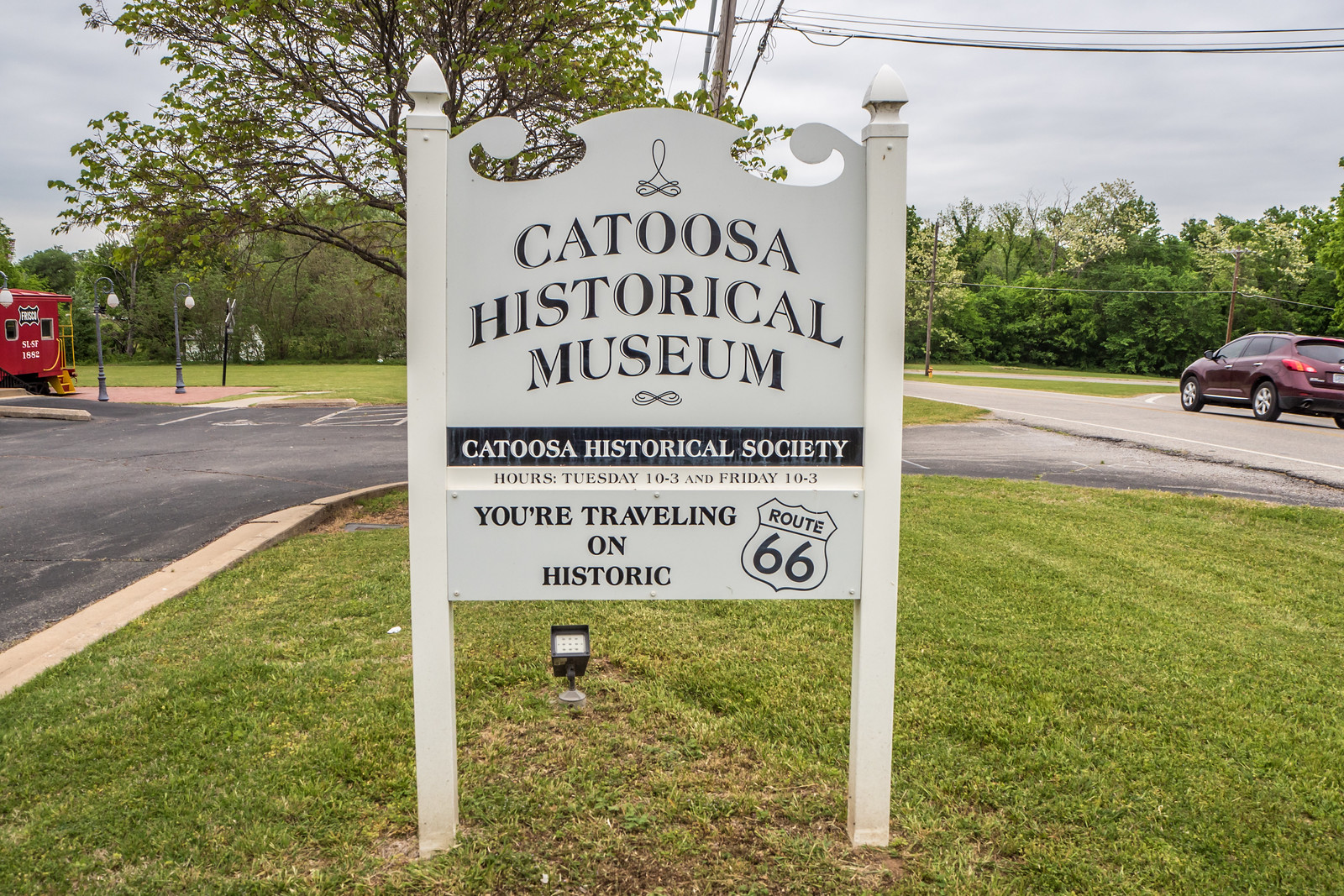The image depicts a white wooden sign positioned in the center of a well-manicured grassy area adjacent to a dark gray parking lot. The sign, supported by two off-white rectangular posts with pointed tops, features a decorative top edge resembling a wave on either side of a bell-shaped middle section. The sky above is light gray and cloudy, contributing to an overcast ambiance.

In the upper part of the sign, in dark blue, all-capital, fancy, curved font, it reads "Catoosa Historical Museum," with what appears to be a symbol resembling an infinity sign and swirl above it. Below this, a black horizontal line divides the sign, beneath which the text "Catoosa Historical Society" appears. Further down, it lists the museum hours as "Tuesday 10 to 3 and Friday 10 to 3" in black text. The bottom section of the sign states, "You're traveling on historic Route 66," with the iconic Route 66 road sign logo beside it.

To the right in the image, a purple car can be seen driving along a gray road in the distance. A thick forest of green trees extends across the background from right to left, and a red railroad caboose is parked in the lot, featuring a yellow stairway possibly as part of an exhibit. Lamp posts resembling old-fashioned gas lights are scattered around the parking lot, which is bordered by another grassy area leading into the tree line, adding to the historical ambiance of the scene.